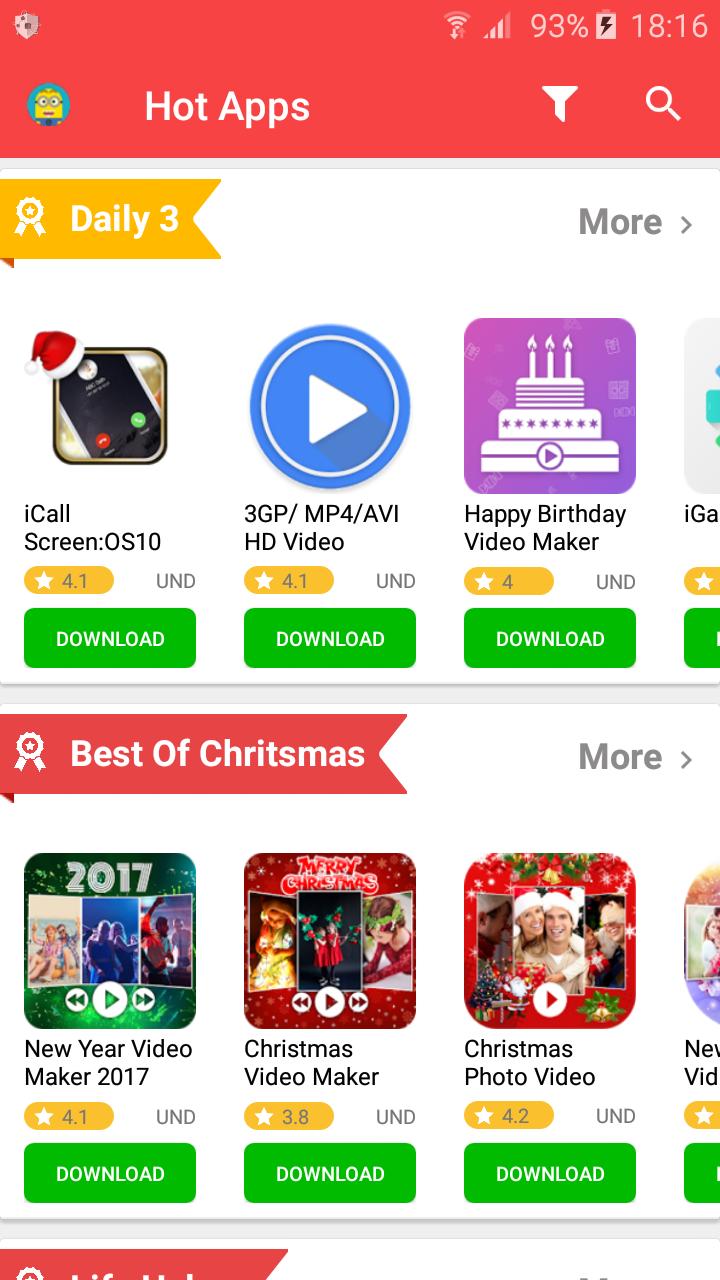This image is a screenshot from a smartphone, documenting a section of an app or website interface. At the top of the screenshot, the device details are visible: the battery life is at 93%, and the time is 18:16. The header of the interface reads "Hot Apps," followed by an orange banner labeled "Daily 3" featuring an award ribbon icon on the left side. On the right side of this banner, it says "More" accompanied by a right-pointing arrow.

Below the header, three app listings are visible:
1. "iCallScreen OS 10," rated 4.1 stars with an available download button.
2. "3GP / MP4 / AVI HD Video," also rated 4.1 stars with a download option under the label "UND."
3. "Happy Birthday Video Maker," which has a rating of 4 stars and a download button labeled "UND."

Following these listings, a red banner with the incorrectly spelled title "Best of Chritsmas," featuring a white award ribbon icon on the left, and "More" text on the right, is visible. Underneath, three additional app listings are presented:
1. "New Year Video Maker 2017," rated 4.1 stars and available for download.
2. "Christmas Video Maker," with a 3.8-star rating and a download option labeled "UND."
3. "Christmas Photo Video," boasting a rating of 4.2 stars with a download button labeled "UND."

At the very bottom of the screenshot, partially cut off, there is another red banner. This image is vertically oriented, being taller than it is wide.